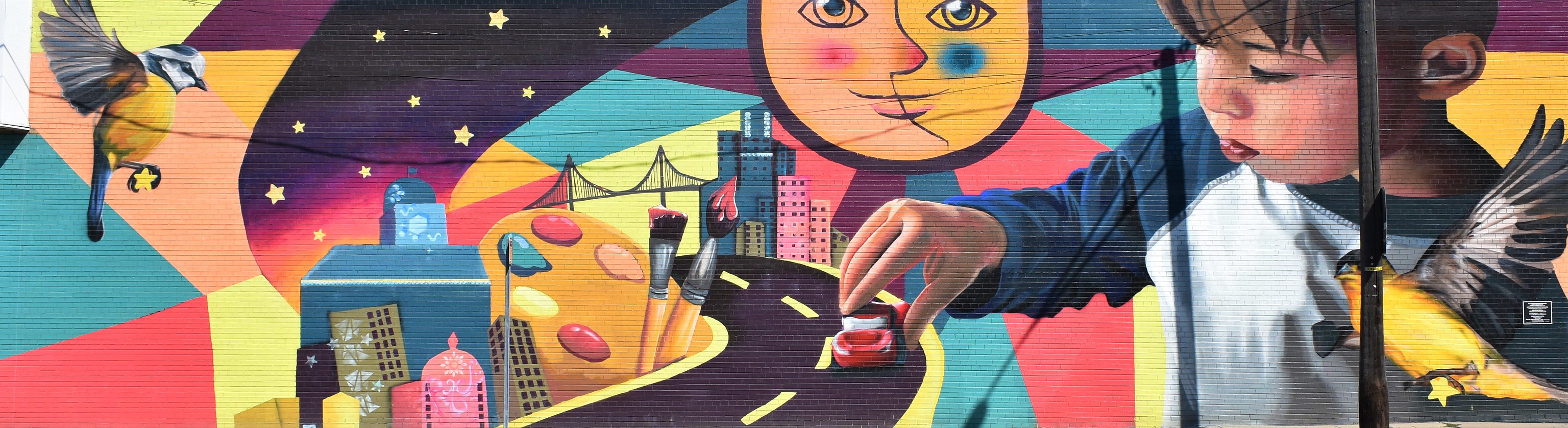The mural is a vibrant, colorful composition with a somewhat abstract-collage aesthetic, painted on a slightly textured brick wall. It prominently features a realistic depiction of a young Japanese boy, possibly a toddler, on the right side. He’s wearing a white and blue long-sleeved shirt and is holding a toy red Matchbox car that is positioned on a cartoon-like black road with yellow dashed lines. Adjacent to this road is an artist’s palette, adorned with paintbrushes smeared with pink paint and containing beige, red, blue, yellow, and pink paints. 

The mural's background is a blend of solid colors including light blue, peach, light red, and yellow, giving it a rainbow-like appearance. There's a section of the background resembling a starscape with a gradient transitioning from yellow at the bottom to orange, pink, violet, and finally black at the top, speckled with little yellow stars. Toward the top center, there's a whimsical face with a pink cheek and a blue cheek, possibly representing a sun or moon, with geometric rays extending outwards. 

On the left side of the mural is a yellow bird with a black and white head and gray wings, holding a small yellow star in its talon. Another similar yellow bird is positioned on the right side, near the boy. Both birds seem to be the same species. Below the face, there’s a depiction of city buildings and a small bridge, adding to the busy yet captivating scenery. This mural, dominated by a mix of cartoon-like elements and juxtaposed with the realistic portrayal of the boy, offers a visually engaging and richly detailed artwork.